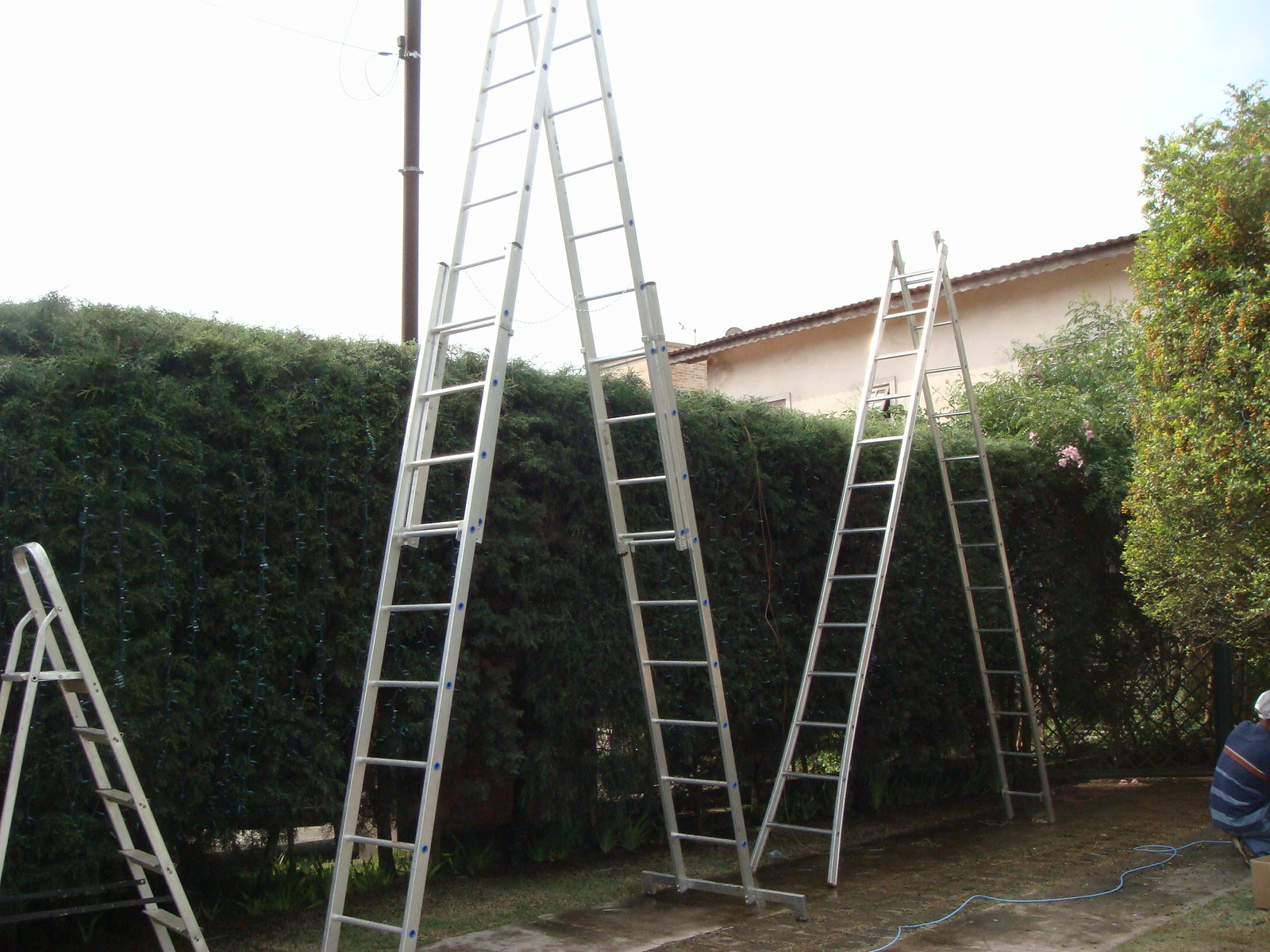In this photograph, three silver metal ladders of varying heights stand in front of a large, dark green rectangular hedgerow. The tallest ladder in the center extends beyond the top of the image, while the ladder on its right reaches slightly above the hedgerow, and the small step ladder on the far left is about half the size of the center ladder. Behind the hedgerow, a mixture of green foliage, including a flowering plant with pink blooms and a large green bush, enriches the scene. To the right, a person is crouching, wearing a distinctive dark blue shirt adorned with white and red stripes and alternating cyan and dark blue sections. A dark brown telephone pole with wires, a partially visible beige stucco house with a brown roof, and a predominantly overcast sky with hints of blue add depth to the background. The ground is a mix of green grass and brown dirt, contributing to the natural setting.